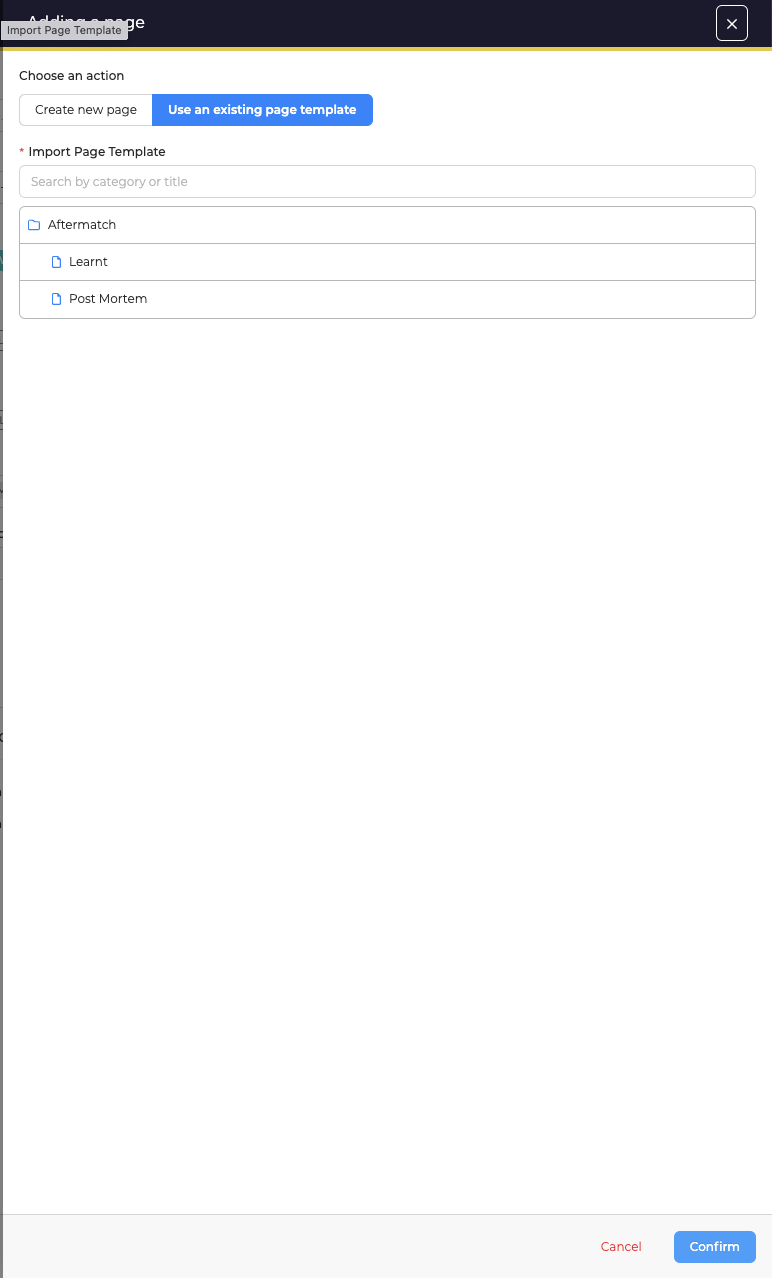The image primarily features a white page with a black banner spanning across the top. The banner's text is obscured by a smaller gray box displaying the message "Import Page Template." On the right side of the black banner, there is a white 'X' inside a square.

Below the banner, black text reads "Choose an action," followed by two adjacent boxes. The first box is white with black text that says "Create a new page." Attached to its right is a blue box with white text that reads "Use an existing page template."

A new row follows, featuring a red bullet next to the black text "Import page template." Adjacent to this is a large gray text box that spans the screen width, stating "Search by category or title."

The subsequent section comprises three outlined rows within a larger box. The first row includes a folder icon and the text "Aftermatch." The second row displays an icon of a piece of paper with the text "LEARNT." The last row features another piece of paper icon alongside the text "Postmortem."

At the bottom right corner of the screen, the word "Cancel" appears in red text, next to a blue box with white text that says "Confirm."